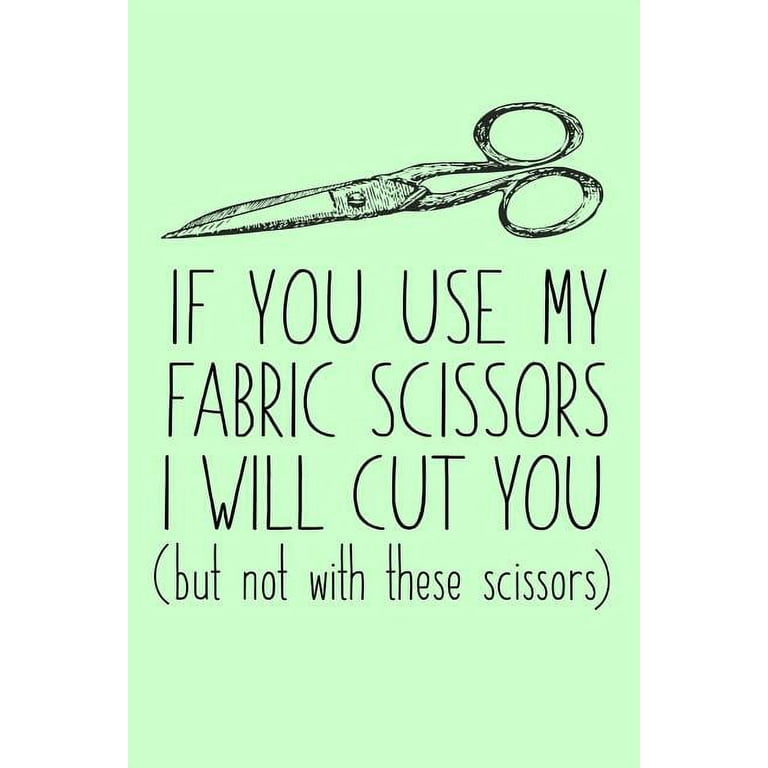The image displays a light mint-green rectangular poster or banner. At the top, there's a black sketch of a pair of fabric scissors with two round handles and sharp blades. Below the scissors, there is a bold, black, uppercase text spread across three lines that reads: "IF YOU USE MY FABRIC SCISSORS, I WILL CUT YOU." Underneath this in smaller, lowercase text within parentheses, it states: "but not with these scissors." The typography is relatively thin with minimal spacing between the letters, emphasizing the humorous yet stern message about the owner's pride in their fabric scissors.